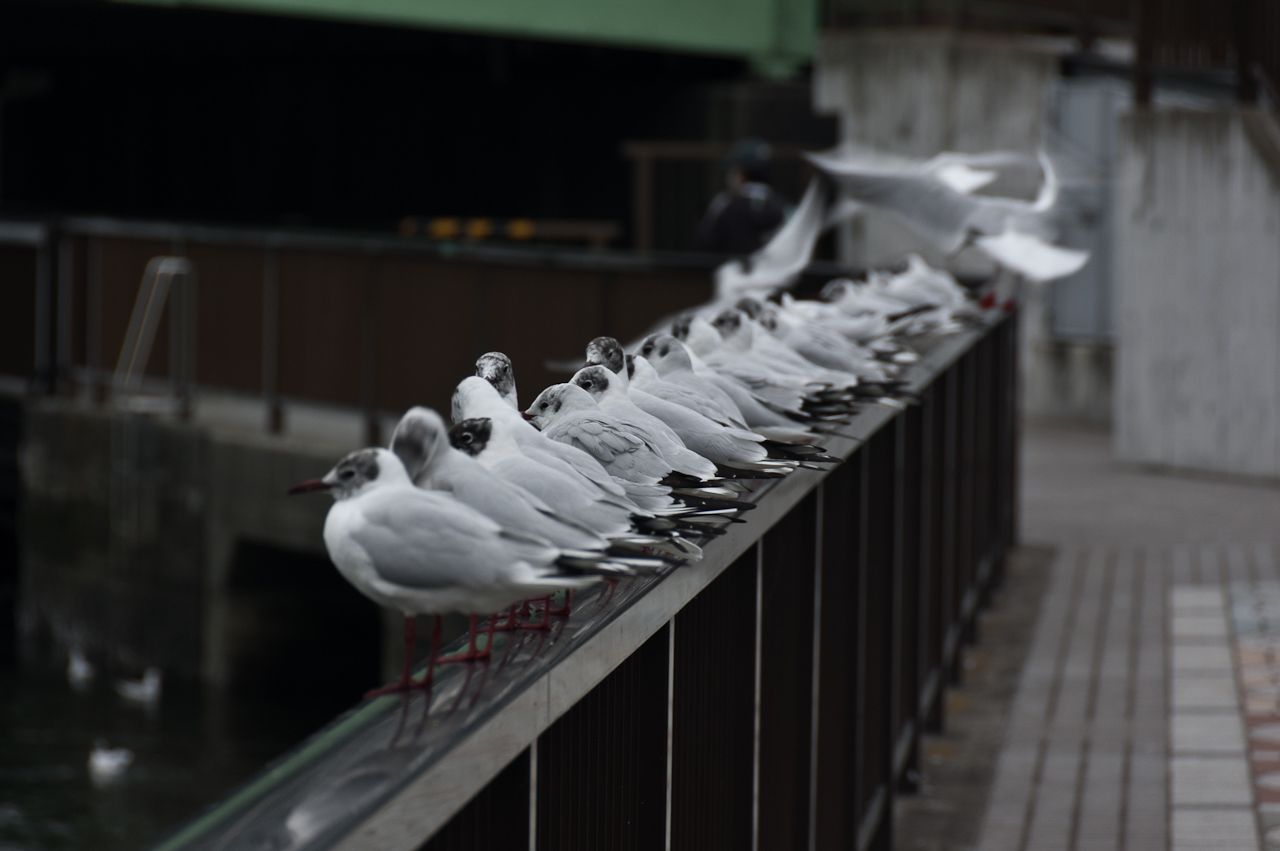The image is a horizontal, landscape-oriented photograph captured outdoors, potentially in a nighttime setting. The background on the left is somewhat dark, suggesting either a building or the night sky. In the bottom left corner, a ladder seems to lead downwards, perhaps into water. The right side of the image showcases concrete walls and a walkway made of concrete blocks and tiles. A black metal hand railing, featuring black supports and a black top, runs diagonally from the bottom left towards the center right and then turns left. Perched along this railing, approximately 20 birds—white and gray with black heads, small black beaks, and possibly black-tipped tails—face to the left. These birds, which could be a hybrid between seagulls and pigeons, are aligned in unison. Some birds are in flight either landing or taking off, but the majority remain perched, seemingly scoping out their surroundings. The walkway below the railing alternates between wooden and stone surfaces, possibly suggesting a harbor setting. The overall scene is tinged with muted colors, contributing to a grayscale-like appearance, amidst a backdrop featuring indistinct shapes and a hint of green from a roof, contrasting with the darker, rustic elements.